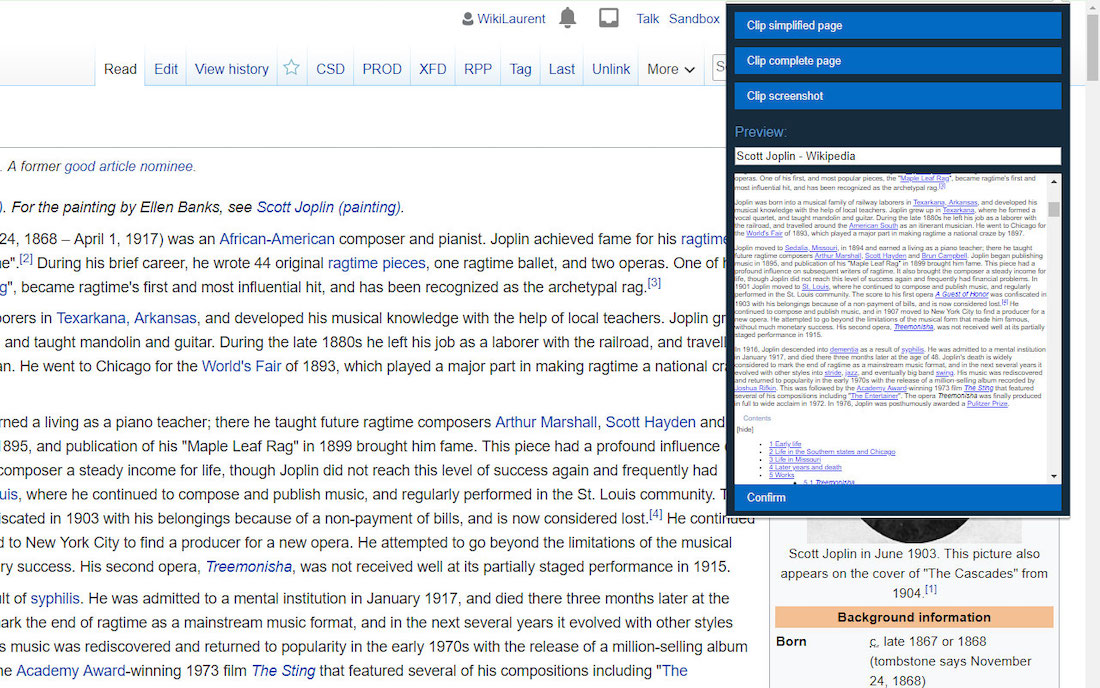This image depicts a screenshot from a Wikipedia-like website, highlighting the user interface elements related to the user "WikiLaurent." Positioned at the top right center of the screen, "WikiLaurent" is accompanied by the "Talk" and "Sandbox" options. A pop-up menu is visible on the right-hand side, featuring several blue buttons labeled as follows: "Clip Simplified Page," "Clip Complete Page," "Clip Screenshot," and "Preview." Below the pop-up menu, the text "Scott Joplin / Wikipedia" indicates that the page being viewed is related to the renowned musician Scott Joplin, suggesting this is indeed a Wikipedia page. The page appears to be a former nominee for "Good Article" status, contributed by user Alan Banks C. Next to the user name "WikiLaurent," there is a profile picture, indicating that this user is currently signed in. The menu options associated with "WikiLaurent" are located at the top left, adjacent to their profile details. This detailed view provides an insight into the navigation and user interaction elements of a Wiki page dedicated to Scott Joplin.